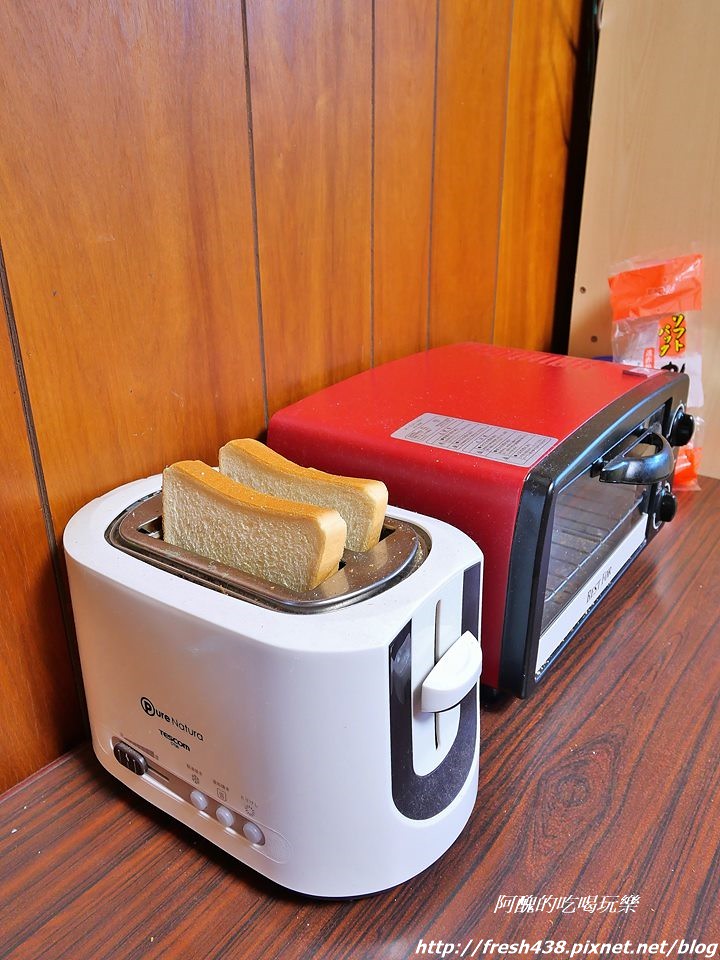The photograph, taken indoors, captures a nostalgic scene reminiscent of the 1970s, characterized by wood-paneled walls. The focal point is a dark brown wood grain countertop, possibly imitation, featuring a collection of kitchen appliances. On the left, there's a white two-slot toaster labeled "Pure Natura" with its distinctive U-shaped silver band and slider handle, holding two pieces of white bread. Adjacent to it is a red and black toaster oven with a glass front, framed in black, complete with round dials and a silver plate displaying directions. Against the wall, there is a clear plastic bag adorned with yellow, black, and orange accents and some Chinese or Japanese text. The scene is illuminated softly, and the bottom right corner of the image displays the URL "http://fresh438.pixnet.net/blog" accompanied by some oriental characters.